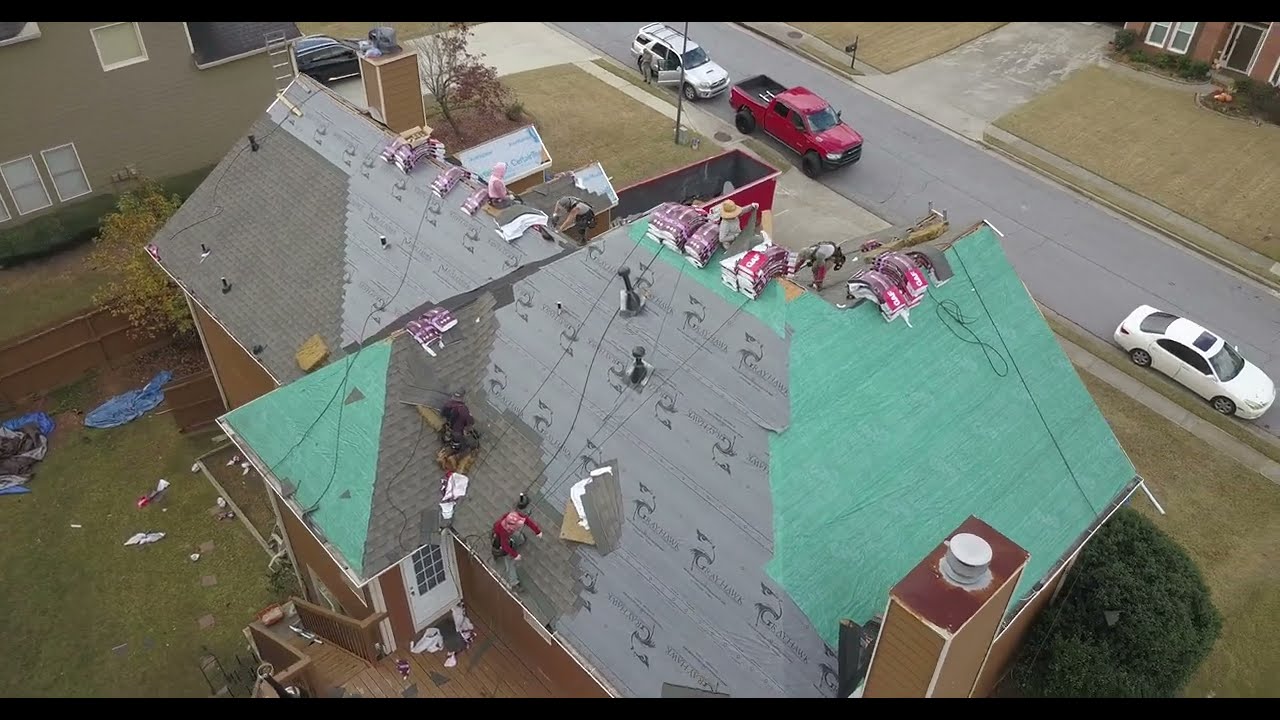This top-down photograph captures a detailed scene of workers actively installing green shingles on the roof of a partially completed, two-story red brick house. The roof, adorned with both green and gray underlayment, features scattered bags of shingles, showcasing the ongoing work. Two chimneys rise from the structure, and a white back door opens to a rear deck. Four men in distinct long-sleeve shirts—red, purple, pink, and gray—are diligently working on the roof. The front of the house borders a small street, where a white car, a red pickup, and a white SUV are parked. In the driveway, a red dumpster sits amid the construction activity. The short green grass in the front contrasts with the backyard cluttered with blue tarps, tools, and debris. Surrounding this scene is a residential neighborhood, visible in the background, hinting at the community setting of this new construction.